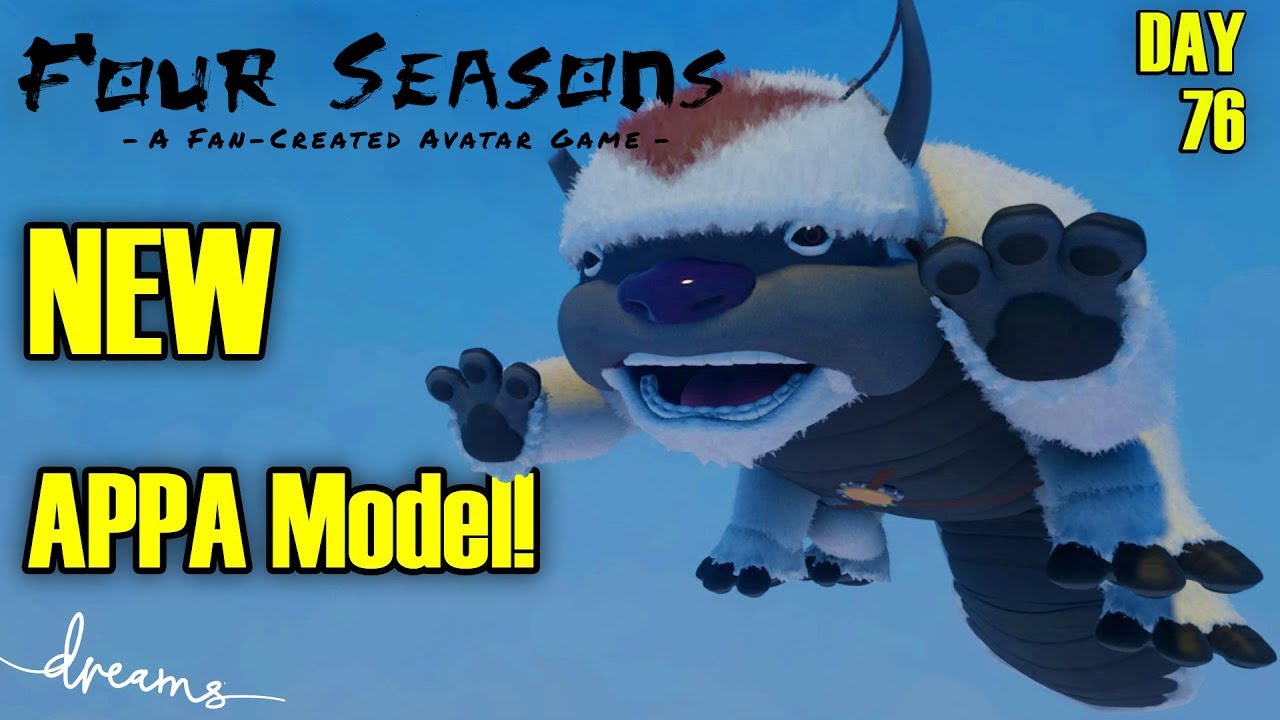This image is a poster for the fan-created avatar game "Four Seasons." The poster is horizontally rectangular, featuring multiple detailed elements and vibrant colors. At the top, in black print, it reads "Four Seasons, a fan-created avatar game." On the right side, a large fantasy animal can be seen, featuring six legs and a Viking knit hat with a red triangle and what appear to be horns. This creature has a gray face, large bulbous black nose, two eyes, and an open mouth with visible teeth. Its body is characterized by blue, gray, and beige tones, giving it a mysterious, almost mythical appearance. The animal's front arms are outstretched, seemingly in a flying or hovering pose, with three fingers on each paw. In the top right-hand corner of the poster, "Day 76" is printed. At the bottom left-hand corner, the word "Dreams" is written in a cursive font above the phrase "New APPA Model!" in bright yellow print.